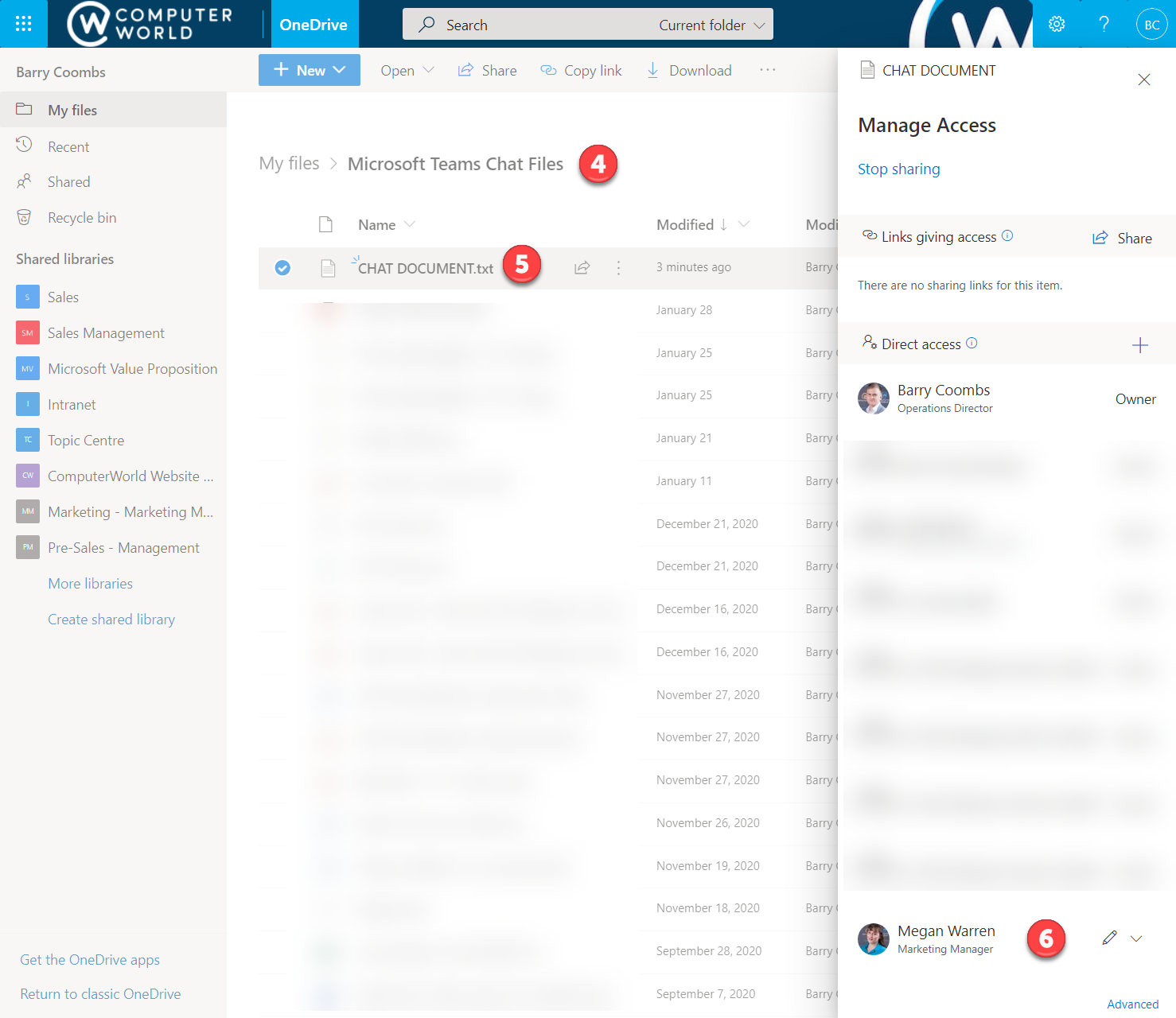In this detailed image, at the very top left, we see the website name "Computer World" prominently displayed. Adjacent to the left of the name is a white "W" enclosed within a white circle. To the right of "Computer World" is the word "OneDrive" set in a blue boxed area, denoting the cloud storage service. Further to the right, there is a search bar that starts with a magnifying glass icon and the word "search" on the left side. On the right side of the search bar, it reads "current folder." 

In the top right corner, there is a circle containing the initials "BC," presumably the user's initials. To the left of this circle are a question mark icon and a gear icon, possibly for help and settings, respectively. Beneath this top right section, we see options like "Chat" and "Documents." 

Further down on the right side, there is a section labeled "Manage access," followed by a blue-highlighted "Stop Sharing" option. Directly beneath, a new section labeled "Giving Access" features a share button on its right.

On the left side of the image, we start with the name "Barry Coombs," followed by a list of categories: "My Files," "Recent," "Shared," "Recycle Bin." Below, there is a section titled "Shared libraries," listing different libraries including "Sales," "Sales Management," "Microsoft Value Proposition," "Intranet," "Topic Center," "Computer World," "Marketing," and "Pre-sales."